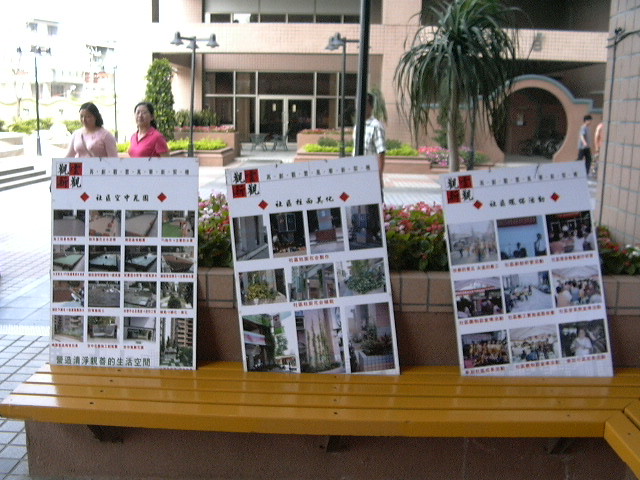This photograph captures an outdoor courtyard scene adjacent to a two-story office building. In the center, there's a wooden bench with yellow horizontal slats, seamlessly integrated into a low concrete wall adorned with a tiled top, forming a planter. This planter hosts a variety of flowers, adding a touch of nature to the urban setting.

Leaning against the bench are three posters, each displaying photographs and text that appears to be either Chinese or Japanese. The contents of these posters remain unclear, possibly being catalogues or calendars. On the left side of the image, two Asian women, one in a pink top and another in a bright pink top, add a human element to the scene. The courtyard features a tile-paved floor, with three to five people walking through it, creating a lively, yet serene atmosphere. In the background, there's a hint of a palm tree, further enriching the setting with a blend of natural and architectural elements.